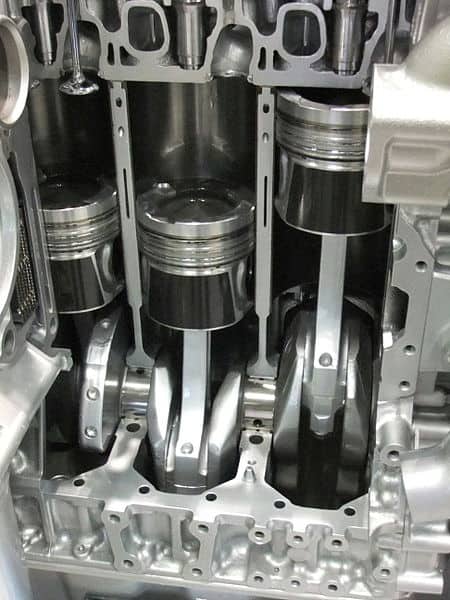The image captures a highly detailed, close-up view of an immaculate and polished engine's internal mechanisms. Dominated by silver, shiny metal and black components, the photograph exhibits three pistons within cylindrical chambers, suggesting motion with two pistons positioned downward and one elevated. The scene, possibly of a demonstrational or newly assembled engine, lacks the usual grime found in typical mechanical environments. Surrounded by drilled holes without screws, the imagery indicates removed or missing covers, providing an unobstructed look at the machinery's inner workings. A distinct rectangular silver box with a steel pipe protrudes out of the frame on the right, adding to the intricate mechanical aesthetic. Despite the ambiguity of the machine's overall function, the captured elements suggest precision engineering, likely made of steel or aluminum, framed within a picture that might be in black and white.